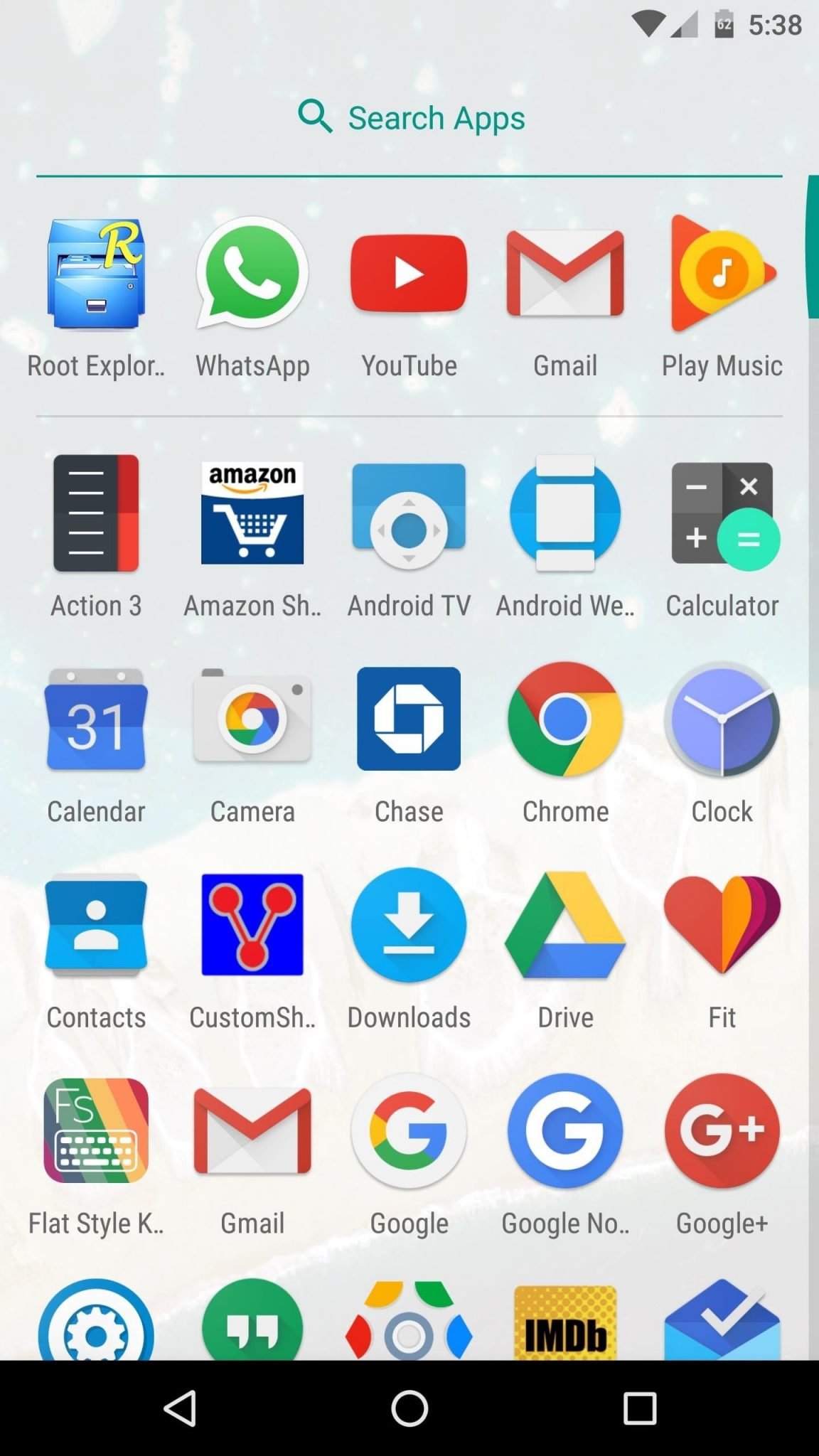An image of a smartphone screen displays various app icons organized in a grid:

- **Status Bar (Top Right)**: 
  - A battery icon with the number "62."
  - A time display reading "5:38," in black.
  - A partially filled signal bar.
  - A fully filled volume bar in black.

- **Search Bar (Middle)**:
  - Turquoise text reads "Search apps" paired with a search icon.
  - A horizontal turquoise line runs left to right beneath the text.

- **Background**: Light gray.

**First Column of Apps**:
1. **Root Explorer**: A blue file cabinet icon with a yellow "R."
2. **WhatsApp**: A green chat bubble outlined in white containing a white telephone icon.
3. **YouTube**: A red square with a white play button (triangle).
4. **Gmail**: An envelope icon outlined in red forming an M shape.
5. **Play Music**: An orange triangle intersecting with a yellow circle containing a white musical note.

**Divider**: A fine gray line separating sections.

**Second Column of Apps**:
1. **Action 3**: A rectangle, brown on the left, red on the right, with white horizontal lines.
2. **Amazon Shopping**: "Amazon" in black with a gold arrow underneath. A white shopping cart against a blue background is at the bottom.
3. **Android TV**: A blue box with a white circle.
4. **Android Web**: A blue circle with a white rectangle.
5. **Calculator**: A gray background featuring minus, multiply, and plus signs; a green circle with two white lines.

**Third Column of Apps**:
1. **Calendar**: A blue square with a white "31."
2. **Camera**: A gray camera icon with the Google colors (orange, red, blue, green, yellow) circled in white in the center.
3. **Chase**: A blue circle containing the Chase Bank emblem in white.
4. **Google Chrome**: A circle divided into red, yellow, and green sections, with a blue center and "Chrome" below.
5. **Clock**: A gray outline with white hands and a blue circle in the center.

**Fourth Column of Apps**:
1. **Contacts**: A blue box, seemingly folded in the middle, with a white person icon.
2. **CustomSH dot dot**: A royal blue box featuring a red antenna icon.
3. **Downloads**: A blue circle with a white download arrow over a line.
4. **Drive**: A triangular icon in green, yellow, and blue representing Google Drive.
5. **Fit**: A red circle partially forming a heart, with segments in orange, burgundy, and pink; labeled "Fit."

**Fifth Column of Apps**:
1. **Flat Style K**: A diagonally striped rainbow background with an "FS" in white and a keyboard icon.
2. **Gmail (repeated)**: Another instance of the Gmail icon, same as before.
3. **Google**: A white circle with a multi-colored "G."
4. **Google NO dot dot**: A blue circle with a white "G."
5. **Google Plus**: A red circle with a white "G+".

**Bottom Section**:
- A black bar with navigation buttons (triangle for back, circle for home, square for recent apps).

**Final Row of Miscellaneous Apps**:
1. **Settings**: Blue outline and white interior with a gear icon.
2. **Chat**: Green chat bubble with white chat icons inside.
3. **Octagon**: Each corner in yellow, green, blue, and red, with a gray center and white interior.
4. **IMDB**: Gold tones with "IMDB" in black text.
5. **To-do**: A 3D blue box in two tones of blue, featuring a white check mark.